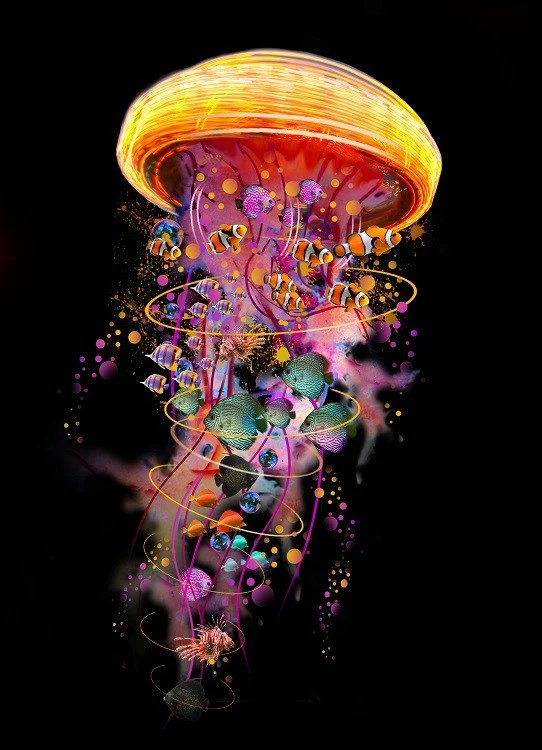A vibrant digital illustration depicts a jellyfish seemingly floating in a dark, almost black ocean. The jellyfish itself is a lively and intricate centerpiece, containing within it a myriad of colorful fish. These fish create a vibrant spiral pattern that extends down the length of the jellyfish, contributing to an energetic and dynamic scene. Decorative circles and a smoke-like effect weave through the illustration, adding to the overall sense of motion and life. The jellyfish's head is adorned with bright yellow hues, while the center underneath glows with a deep, rich blend of red and almost purple tones.